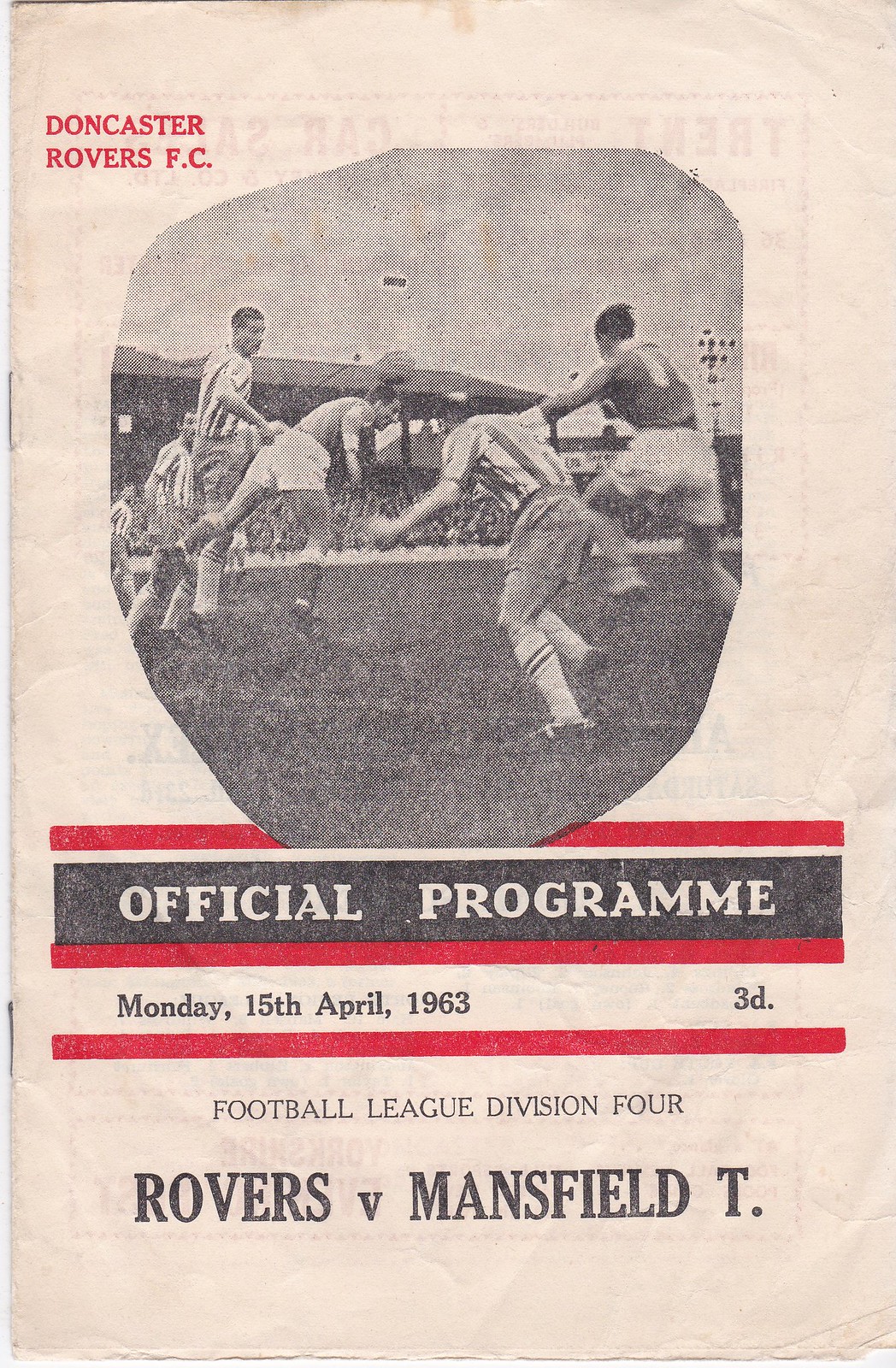The image shows the cover of an old soccer program, aged and printed on thin, off-white paper. At the top left, "Doncaster Rovers FC" is printed prominently in red. Below this is a misshapen oval containing a black-and-white photograph of four soccer players jumping to head the ball during a match. The oval reveals that the paper is so thin you can somewhat see through to the other page. Below the photo, two red lines sandwich a black rectangle with the white text "Official Program." Further down, in black font, the details read "Monday, 15th April 1963, 3D" with an additional red line underlining the date. Lastly, a small black font denotes "Football League Division 4," and underneath in larger bold black capitals, it announces "Rovers vs. Mansfield T." The aging paper is held together on the left side by two staples.